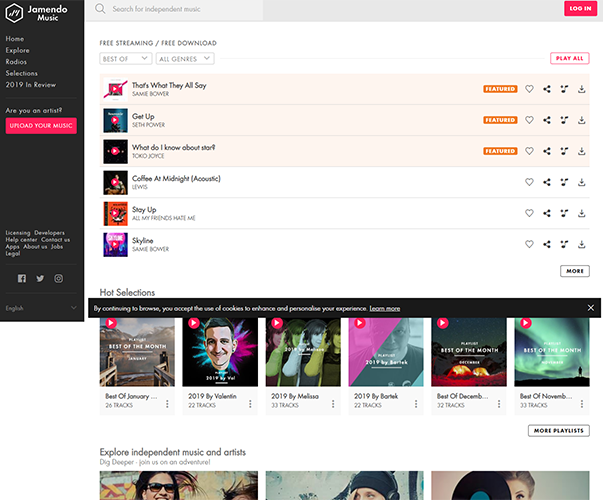This is a descriptive and detailed caption for the given image:

---

The web page for Jamendo Music, an independent music platform, is intricately laid out with a range of options for users. On the far left, there is a vertical navigation bar in black, containing five tabs: "Home," "Explore," an unidentified tab, "2019 in Review," and a tab asking, "Are you on Earth?" Below these, the option to "Upload your music" is prominently displayed. Social media links for Facebook, Twitter, and Instagram are also included in this section.

Central to the layout is a search box labeled "Search for independent music," helping users easily discover new tracks. To the far right, users can log in to their accounts. Beneath this, there are options for "Free Streaming / Free Download," a drop-down menu for "Best Of," another for "All Genres," and lastly, a "Play All" button for immediate playback.

The main content area features several sections highlighted from top to bottom. Featured tracks include "Get Up" by Seth Power. However, other tracks, such as "What Do I Know About...," "Coffee At Midnight Acoustic," "Stay Up," "All My Friends Hate Me," and "Skyline" by possibly "Same Bomer," are mentioned with some uncertainty about the group names or titles due to readability issues.

Further down, the site showcases "Hot Selections," featuring albums like "Best Of Journey," "2019" by Valoran, and another "2019" album from an unreadable artist name. There are also "Best Of" listings for December and November. At the bottom of this section, a cut-off area teases more content under the heading "Explore Independent Music and Artists," along with displayed photographs and album covers. Below these album covers, independent artists are featured, offering a glimpse into the rich diversity of content available on Jamendo Music.

---

I hope this better captures the detailed layout and elements of the Jamendo Music web page.